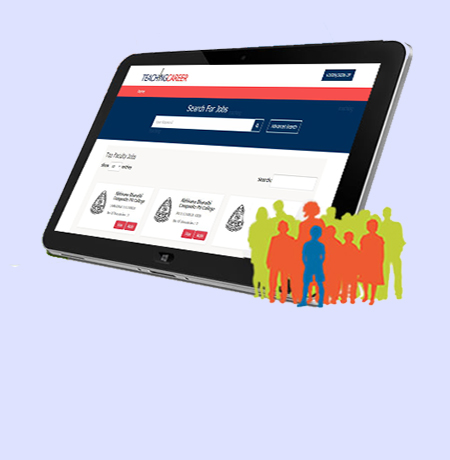The image showcases a tablet displaying a website related to teaching careers. The website interface is framed by a white bar at the top, followed by a red bar below it. On the white bar’s upper left section, the title "Teaching Career" appears, with "Teaching" written in black or blue and "Career" in red. Adjacent to this, on the right, is a blue button that is indistinguishably blurry.

Directly below this section, on the left side of the red bar, is white text that potentially represents a home button. Underneath this bar is a blue box containing the text "Search for jobs" next to a search bar and a magnifying glass icon. Farther to the right, another blue button appears, though its text is too blurry to discern.

The main content under these bars features a white background displaying three silver-colored items, each accompanied by a red button beneath them. Additionally, in the bottom right corner of the tablet, outside the screen, there are silhouettes of green, orange, and blue human figures.